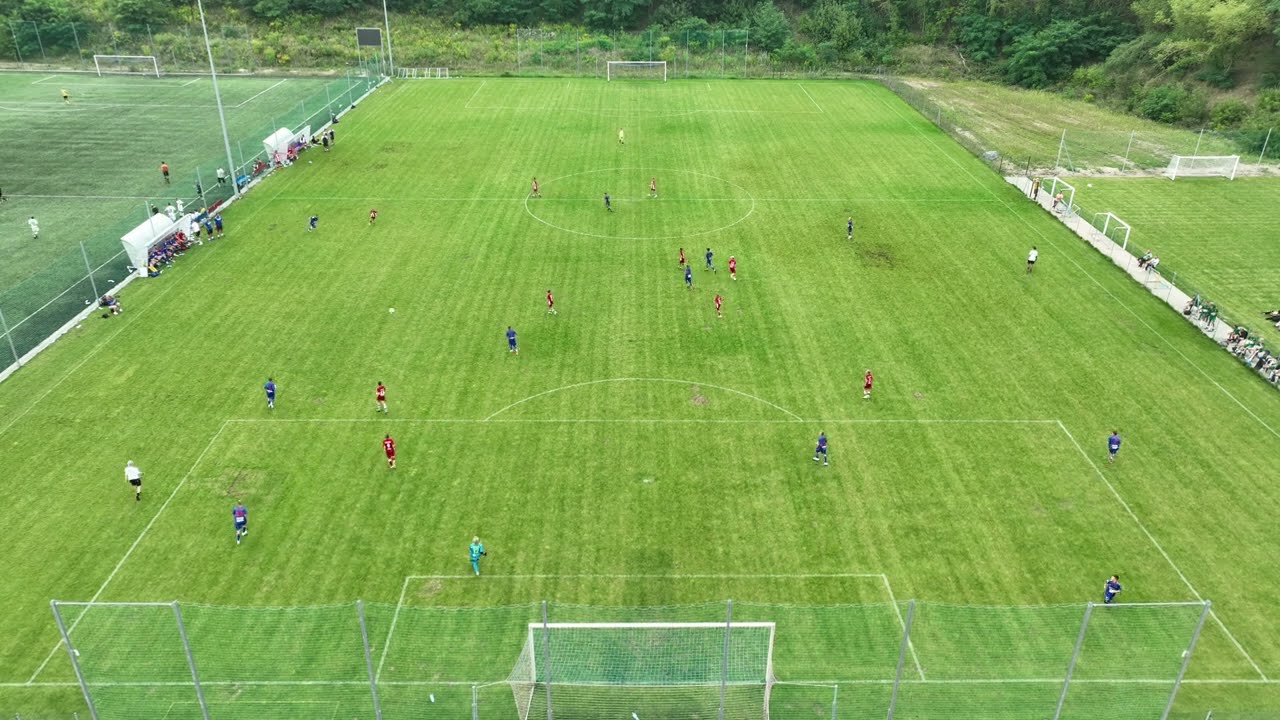The image captures an aerial view of a well-manicured soccer field taken from about 40-50 feet above and behind one of the goals. The field is clearly marked with white lines, and there's a game in progress featuring two teams: one in red and white uniforms and the other in blue and white. The blue team's goalie is distinguishable by a light aqua-colored outfit. Scattered along the sidelines are a few spectators, particularly concentrated towards the right. On the right side near the top of the image, there appears to be an additional goal area, possibly used for practice or a smaller field. To the left in the upper part of the image, another adjacent soccer field can be seen with additional players on it. The background is adorned with a hill covered in bushes and trees, adding a natural frame to the lively scene.